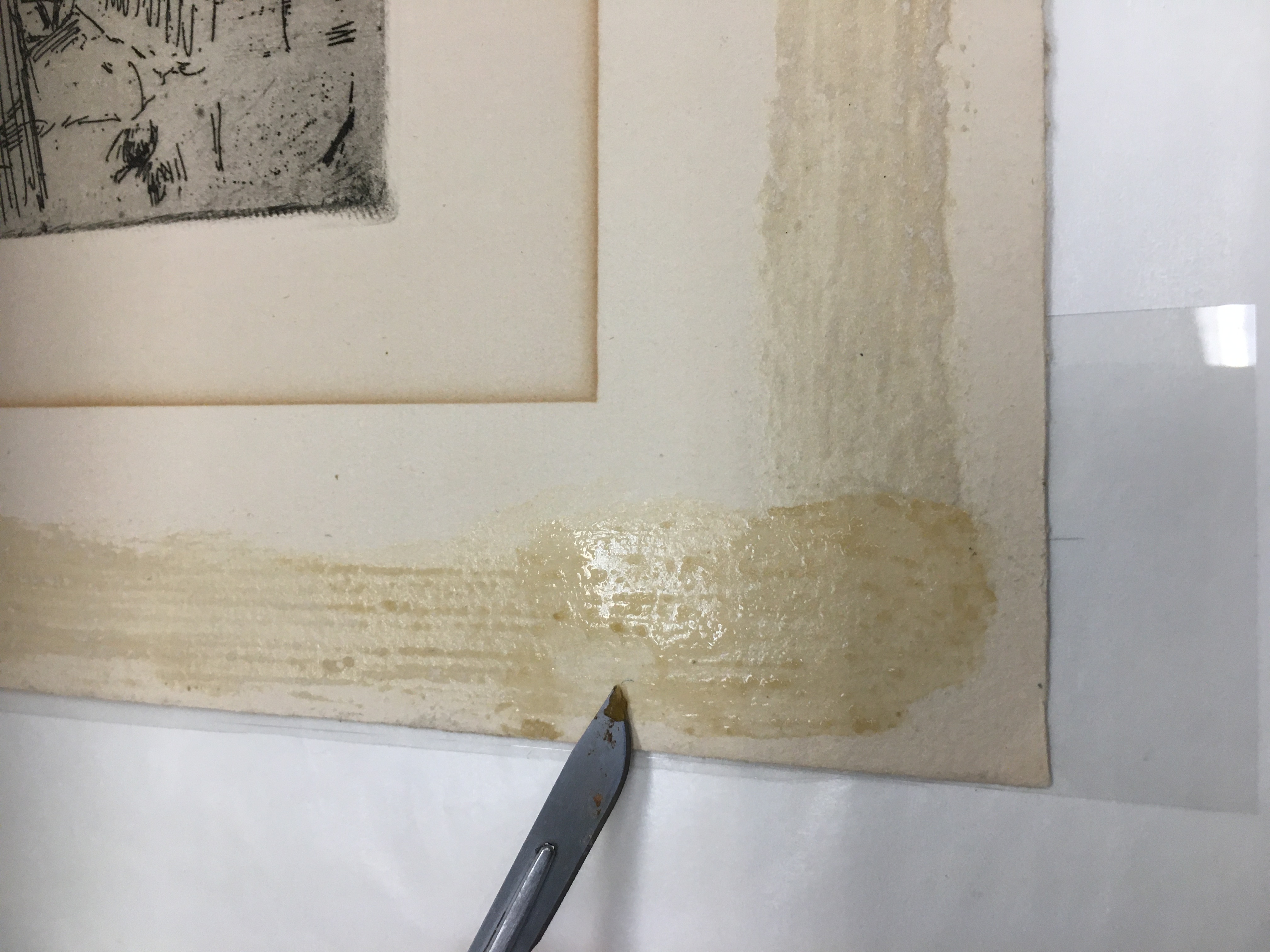This close-up photograph captures the partially repaired back of a matted black and white print. The print rests on a light beige or cream-colored canvas that appears to have been recently unframed, as evidenced by glue marks around its edges. On the left side, there's a smaller square piece of gray paper adorned with black lines in no particular shape, with one blotch almost resembling a person. A silver instrument, likely an X-Acto knife, is seen near the edge of the mat, possibly smearing the wet glue along the sides. The background features a big light gray wall, a glimpse of a white wall, and what seems to be a small metal scaffold near the bottom. The entire setup is partly obscured by a piece of square glass.